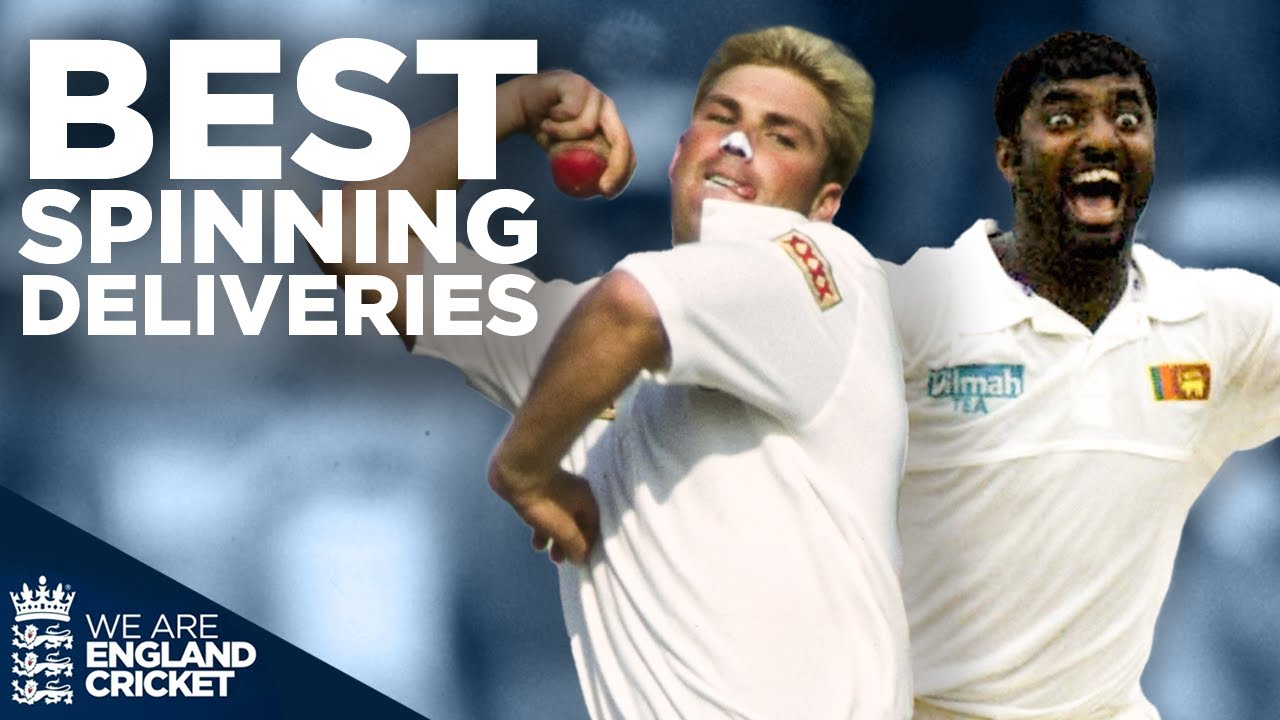The image is a vibrant advertisement for cricket, showcasing two players prominently on the right side against a blurred blue background. At the top left corner, "Best Spinning Deliveries" is written in bold white block letters. In the lower-left corner, the England Cricket logo features a crown atop three heraldic lions, accompanied by the slogan "We are England Cricket."

The two players bring the ad to life with their dynamic postures and expressive faces. The player on the left, a white man with blonde, slicked-back hair, has his arm pulled back, poised to throw a cricket ball. He dons a white jersey with four 'X' marks on the shoulder and sports tape on his nose. The player on the right, an Indian man with black hair and facial hair, is jubilantly yelling with his arms wide open. His white shirt features the name "Dilma T" and a small flag. Both players display intense energy, capturing the excitement and passion of the game.